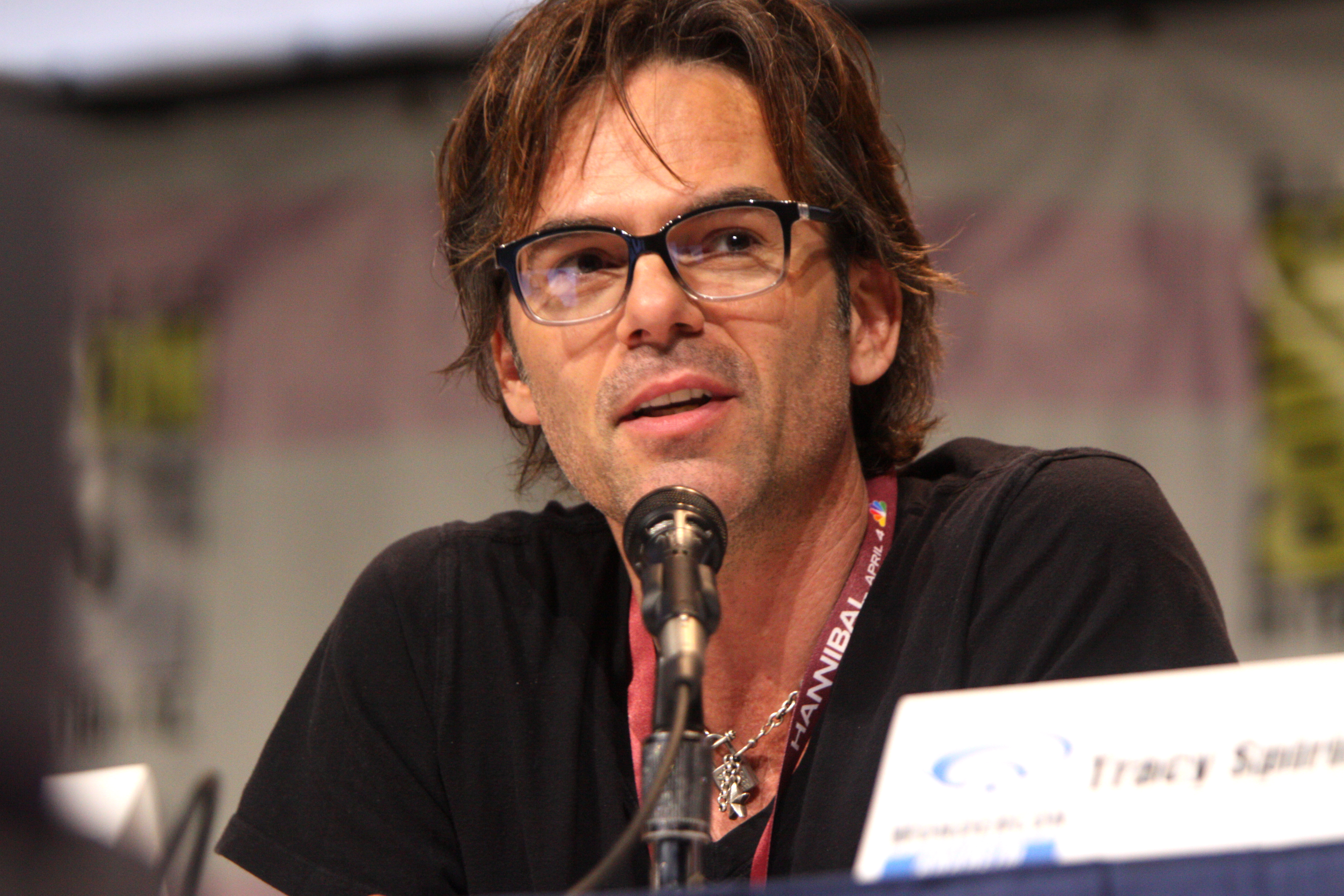This photograph captures a close-up of a man who appears to be a panelist at a convention. The setting includes a panel table with a blurred background, possibly a tent with white drapes and a wide pink stripe. The man, a white male, is likely in his late 40s to early 50s. He has dark brown hair featuring red highlights that is somewhat long and messy around his face, reminiscent of a rock star's style. His eyes, described as soft and gentle, enhance his attractive appearance. He is clean-shaven and wears black-rimmed glasses with transparent bottoms. He is dressed in a black or brown t-shirt, accessorized with a silver or gold chain, and a red lanyard featuring white writing, likely holding a convention name tag. The man is engaged in speaking or answering a question, directed towards his left. A black microphone is positioned in front of him, and there is an unreadable white sign on the table to his left shoulder.